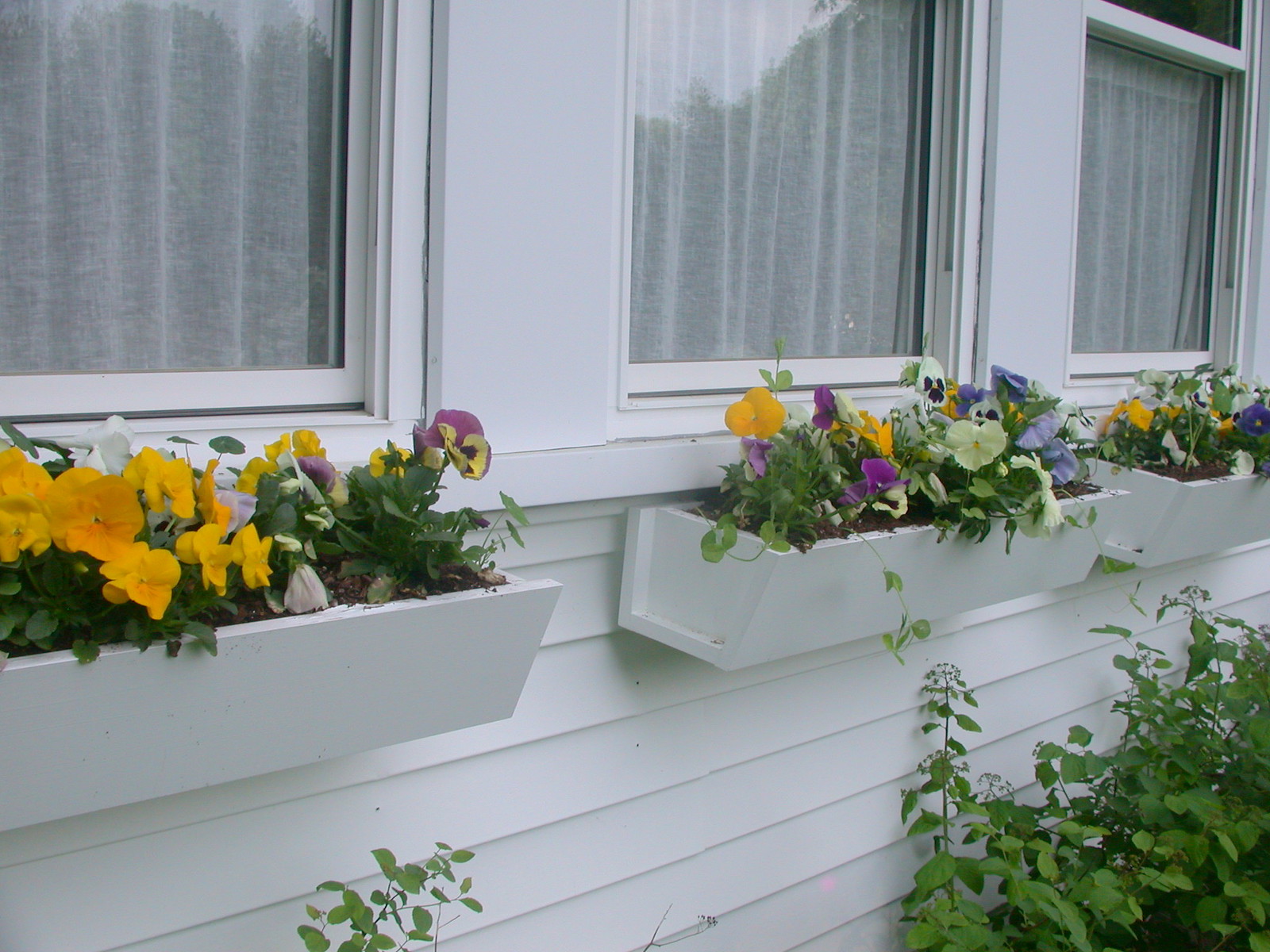The image depicts the outside wall of a white house with three equally spaced windows adorned with white sheer curtains covering the bottom halves. Each window has a matching white planter box filled with a vibrant mix of flowers: yellow blooms with round petals, small white flowers with purple centers, and solid purple flowers. The flower boxes contain a similar arrangement of these flowers, with varying proportions of each color. The windows reflect some sunlight and the tree line behind the viewer. Below the flower boxes, there are small, leafy plants reaching upwards. The house features a tiled exterior and captures a scene on what seems to be an overcast day or a side of the house in the shade, giving it a tranquil, inviting appearance.